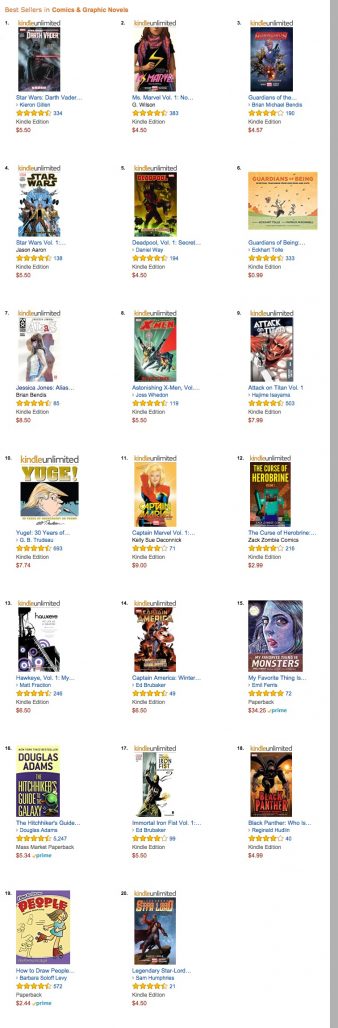This vertical image, likely accessed from a computer or smart device, features a white background that seems to be borrowed from the user’s screen rather than being an independent color. In the top left corner, text in orange reads "Bestsellers in Comics and Graphic Novels." The image lists a series of bestsellers, each accompanied by a number, a thumbnail image, a title, the star rating, the number of reviews, the edition type, and the price. The items are organized in rows: 1 to 3 on the first row, 4 to 6 on the second, continuing sequentially until the final row, which lists items 19 and 20. A gray bar is visible along the right-hand side of the image.